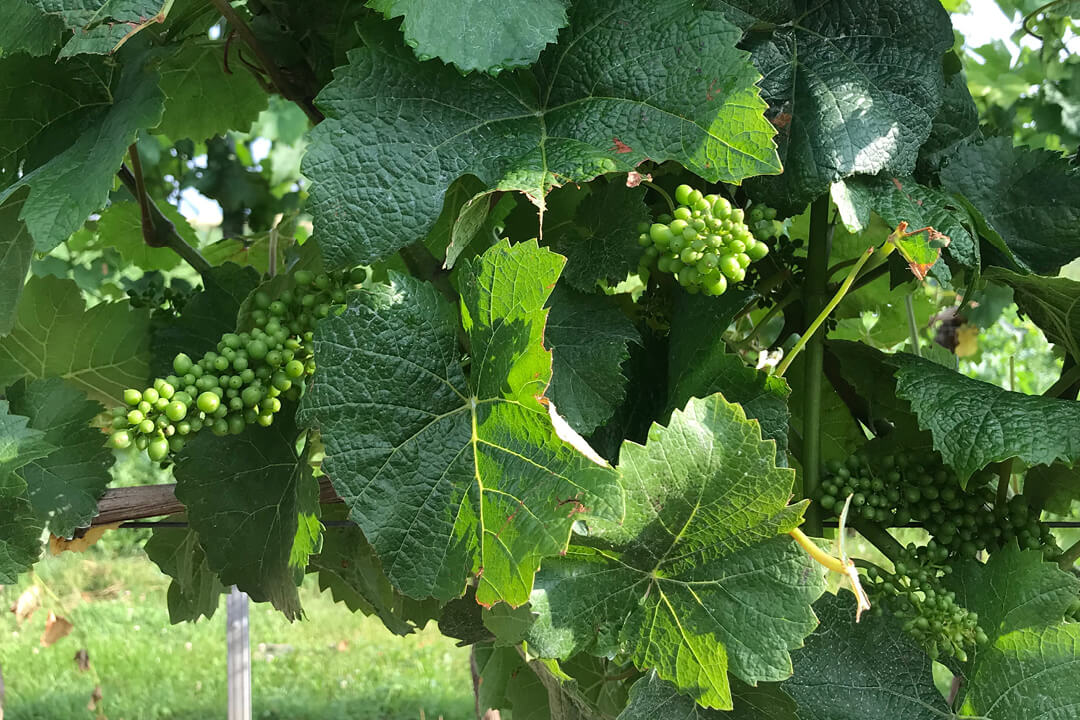In this detailed garden photograph, we observe a vibrant scene dominated by broad, verdant leaves, possibly belonging to a vine plant. These leaves, reminiscent of blackberry foliage yet without the characteristic thorns, create a lush foreground. Nestled among them are clusters of greenish-white berries with delicate spots of pink near their centers, resembling early-stage grapes. The clusters, interwoven with wooden stems, appear to gleam slightly in the light.

In the lower left-hand corner, a patch of blurry grass, interspersed with small brownish leaves, provides a soft, earthy contrast. Sunlight filters gently through the upper right-hand corner, casting a dappled glow that intermittently illuminates the leaves, highlighting their intricate veining. Central to the composition, one leaf is notably half-lit, its right side bathed in sunlight while the left remains in shadow. The photograph exudes a serene, almost timeless quality, with the gentle play of light and natural elements evoking a peaceful garden setting.